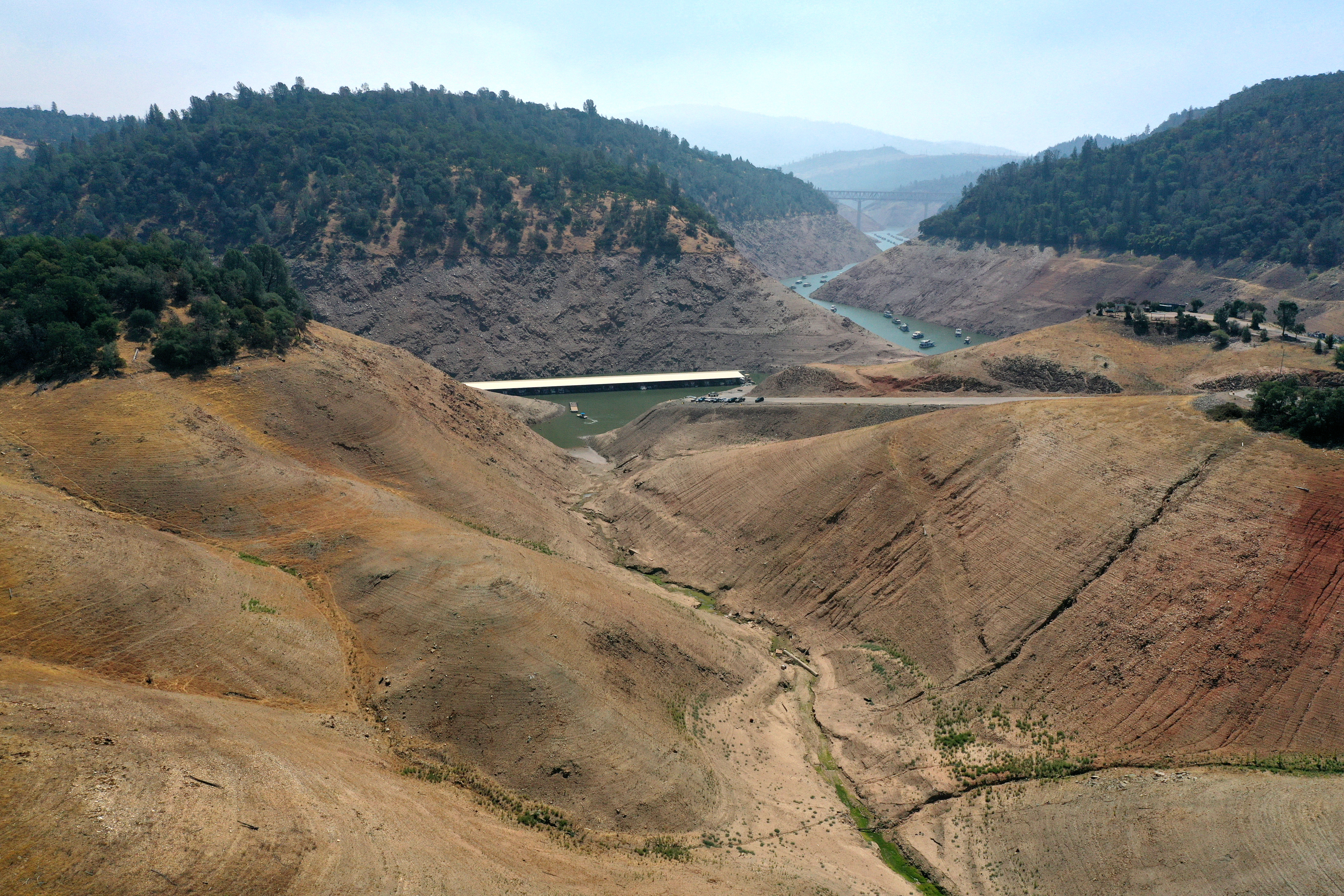In the image, a vast plain stretches out before you, primarily covered in dirt with sparse patches of grass. The terrain consists of a series of rolling hills, framed by two distinct bodies of water—a lake and a river—separated by a narrow strip of land. One body of water exhibits a rich blue hue, while the other takes on a greener tint. In the far distance, a bridge arches gracefully, providing a pathway from one hill to another. Below the bridge, the bluish waters shimmer under the light, transitioning to green in certain sections. As your gaze moves further back, the landscape becomes more densely forested, with trees dotting the horizon. The sky above is a light blue, adorned with a few white clouds and an overall foggy ambiance. Near the green-tinted water, there appears to be a wooden dock or platform, suggesting a place where one could walk across or simply pause to take in the serene surroundings.